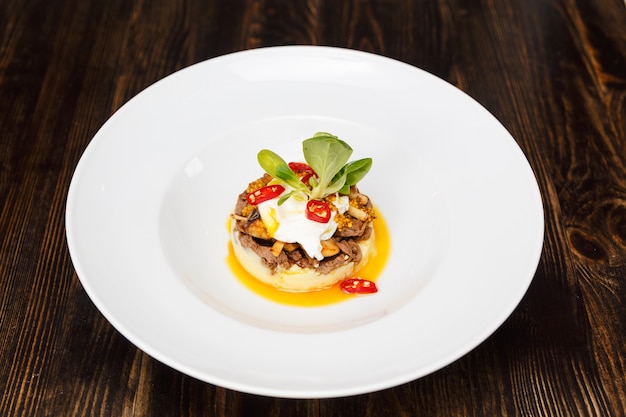The image features a white bowl or plate set on a dark wooden table. Inside the dish, the food is arranged in layers. The bottom layer appears to be a yellow, runny yolk or sauce. Above it, there is a cream-colored substance which might be fish or another sauce. This is followed by a brown layer that could be crumbled meat, possibly chicken or hamburger. On top of that, there's another white layer, potentially sour cream, adorned with scattered slices of red tomatoes or peppers. Finally, garnished on the very top are some green leaves, and possibly pieces of pasta or corn. The intricate layering and minimalist portion suggest it could be a creation from a fine dining establishment, emphasizing artistic presentation.